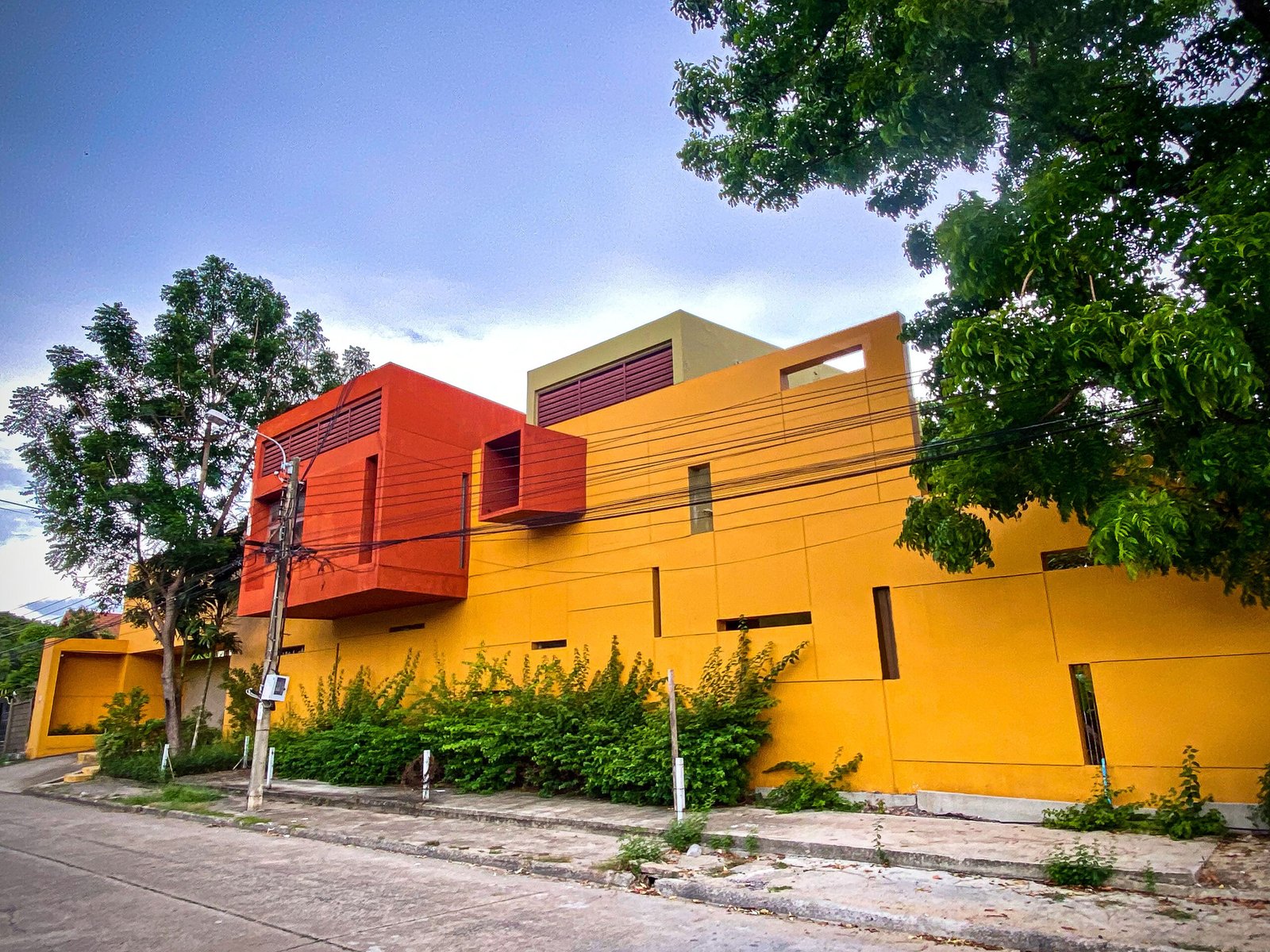This landscape-oriented exterior photograph captures a vibrant and complex building façade composed of modular cubical components with a geometric, almost architectural mosaic design. The dominant structure features a prominent yellow wall, meticulously assembled from various rectangular pieces aligned at right angles, creating a visually striking grid of horizontal and vertical openings. Two orange cubical elements protrude from the wall, one of which displays a grill, adding to the architectural intrigue. 

At street level, green overgrown bushes line the front of the building alongside a sidewalk. Edging the scene, a tree with lush, bright green leaves extends into the upper right-hand corner, adding a natural contrast to the angular constructions. The street, visible in the bottom left, appears aged and grey, contributing to the urban setting, while a light pole with numerous electric wires stands in the left-hand corner, intersecting the scene.

Above and behind the yellow structure, a pale gray rectangular building with a front-facing grill emerges, hinting at a larger complex. The backdrop of the image presents a clear blue sky with wisps of clouds, completing this detailed exterior view of a notably colorful and architecturally intricate street-side building.